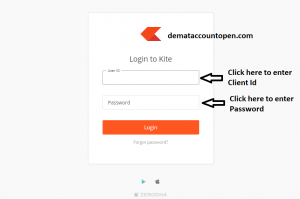The image appears to be a screenshot taken from a computer, centered on a horizontal, light gray rectangular background. Within this background, there lies a smaller white vertical rectangle positioned centrally.

At the top center of this white rectangle, there is an orange arrow pointing left. Beside this arrow, partially extending into the gray area, is the black text "Demataccountopen.com." Beneath this text, it says "Log in to Kite" in black font.

Below this heading, there are two input fields: one labeled "User ID" for entering the username, and another labeled "Password" for entering the password. Near the bottom of the white rectangle, there is an orange login button labeled "Log In." Below the login button, a link says "Forgot password."

On the right side of the white rectangle, extending slightly into the gray area, there is an instructional black text. An arrow pointing towards the "User ID" field reads "Click here to enter a client ID," and another arrow pointing towards the "Password" field reads "Click here to enter password."